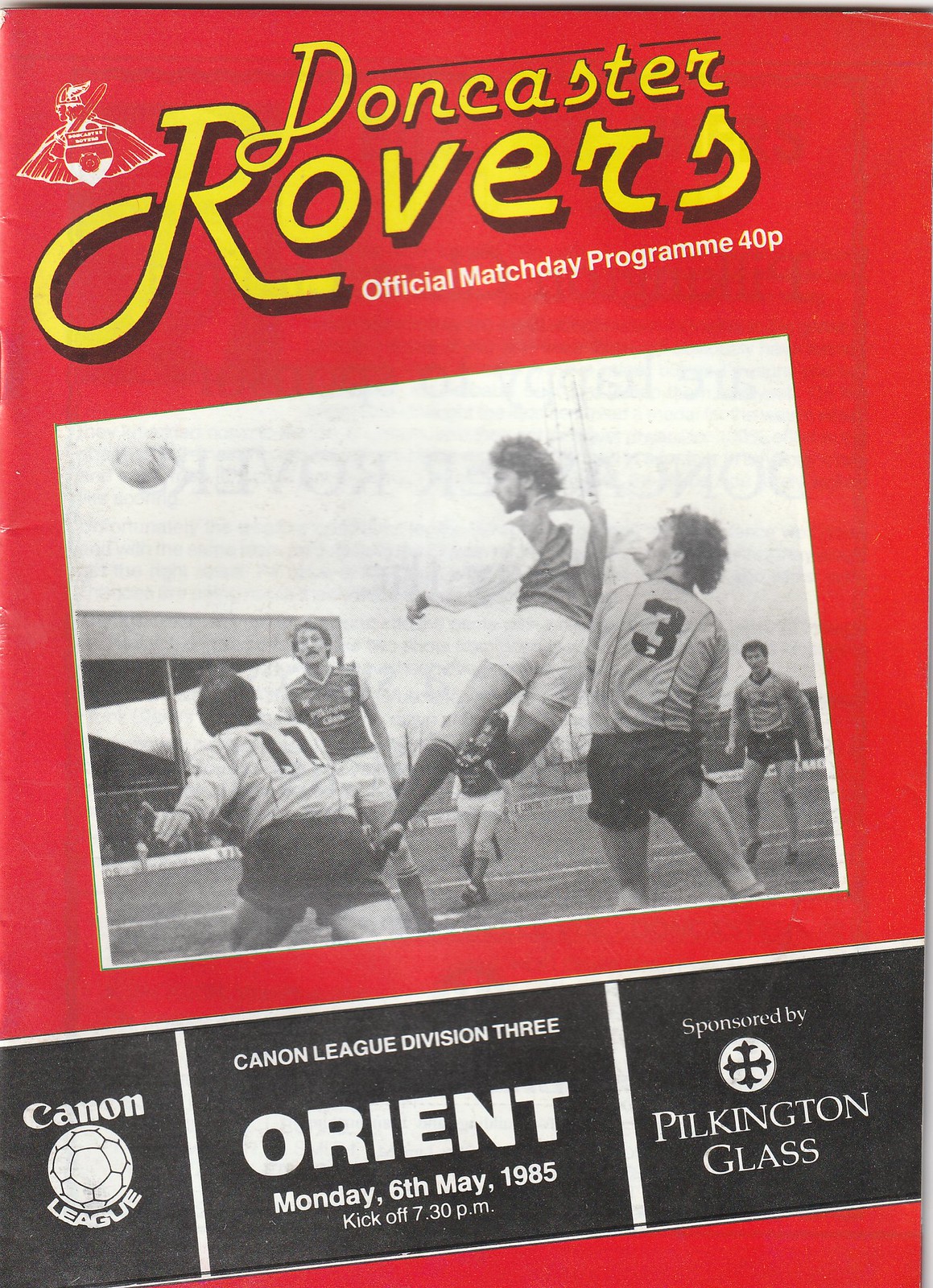The cover of the Doncaster Rovers official Match Day Program, priced at 40 pence, is predominantly red with a striking yellow title. Below, in white text it states, "official match day program." The centerpiece of the cover features a black and white photograph capturing the intense action of a soccer match. In the photo, a player, wearing the number 7 jersey, leaps into the air, seemingly executing a header with teammates and opponents, including players in jerseys number 11 and 3, surrounding him in the stadium. A black diagonal banner runs from the bottom left to above the right corner, with three panels featuring white text. The left panel reads “Canon League,” accompanied by a soccer ball logo. The middle panel details “Canon League Division III, Orient,” and the date and time of the match, “Monday, 6th of May, 1985, kickoff at 7.30 p.m.” The right panel extends the information, “sponsored by Pilkington Glass.”